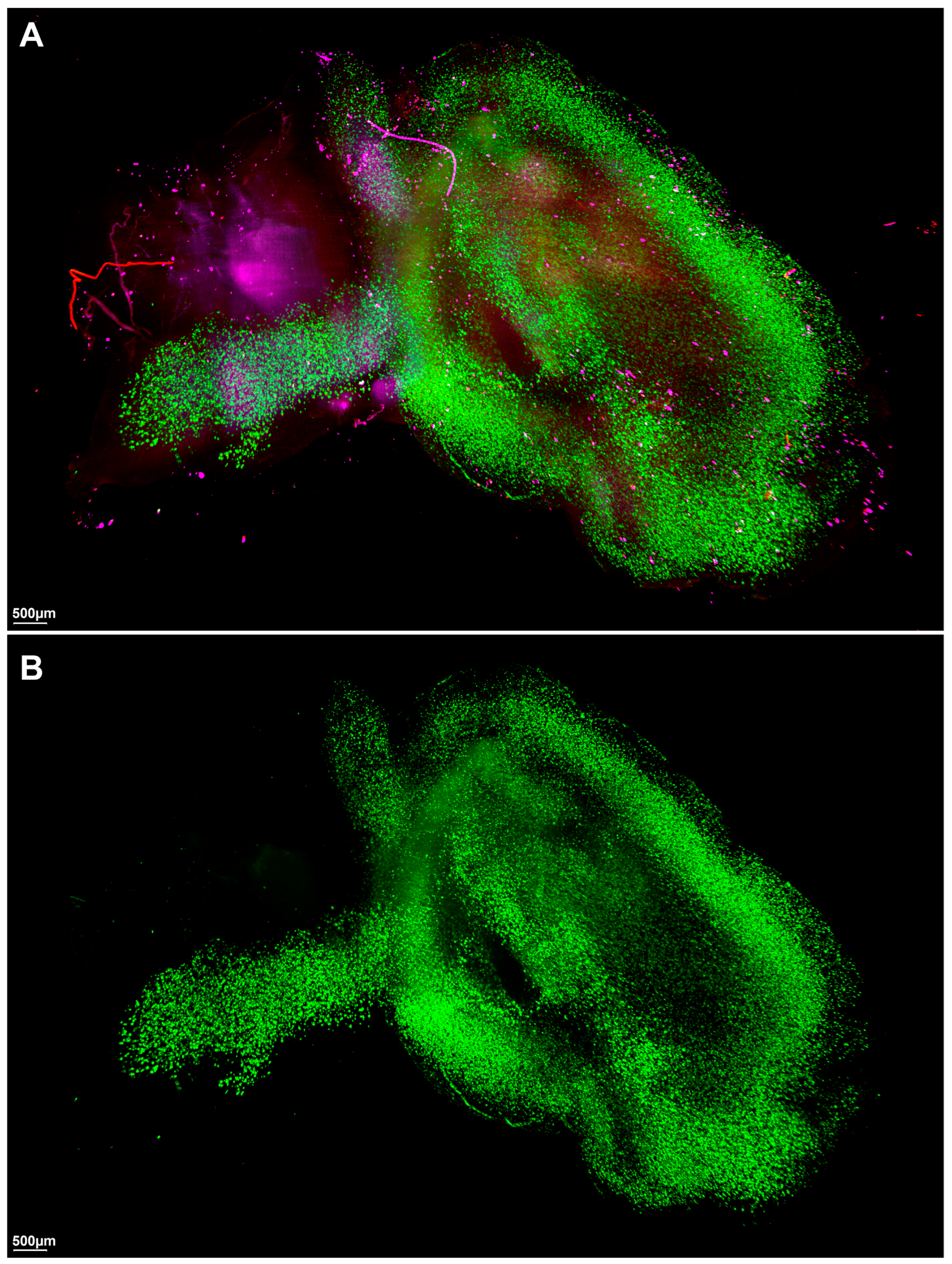The image comprises two panels labeled A (top left) and B (bottom left), each with a 500-micrometer scale. Both panels feature a dense array of tiny, bright green dots against a light purple, almost black background. Panel A exhibits an intricate design with bright green speckles and a scattering of fuchsia, pink, and red dots, appearing almost mist-like. Some viewers noted the suggestion of a face in the pink areas. In contrast, Panel B displays a similar pattern of bright green dots but lacks the pink and red hues seen in Panel A. Both panels include a name or text in the bottom left corner, though it is too small to be legible. The overall impression is of highly detailed, possibly computer-generated images resembling a microscopic or molecular perspective.